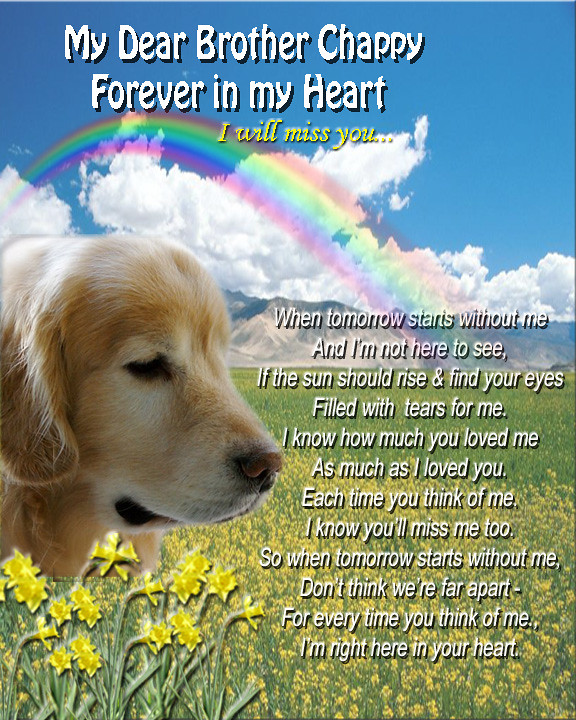The image is a memorial poster for a dog named Chappy. It features an older golden Labrador retriever, visible only from the neck upwards, with white markings around its mouth. The dog is positioned on a digitally edited background showcasing a serene field of yellow flowers, with mountains in the distance under a bright blue sky filled with white clouds. A rainbow arcs gracefully above the dog's head, enhancing the poignant atmosphere. The heartfelt text on the poster reads: "My dear brother Chappy, forever in my heart, I will miss you. When tomorrow starts without me, and I'm not here to see, the sun should rise and find your eyes filled with tears for me. I know how much you love me as much as I loved you. Each time you think of me, I know you'll miss me too. So when tomorrow starts without me, don't think we're far apart. For every time you think of me, I'll be right here in your heart." The poignant message accompanies the touching visual elements, creating a loving tribute to the beloved pet.